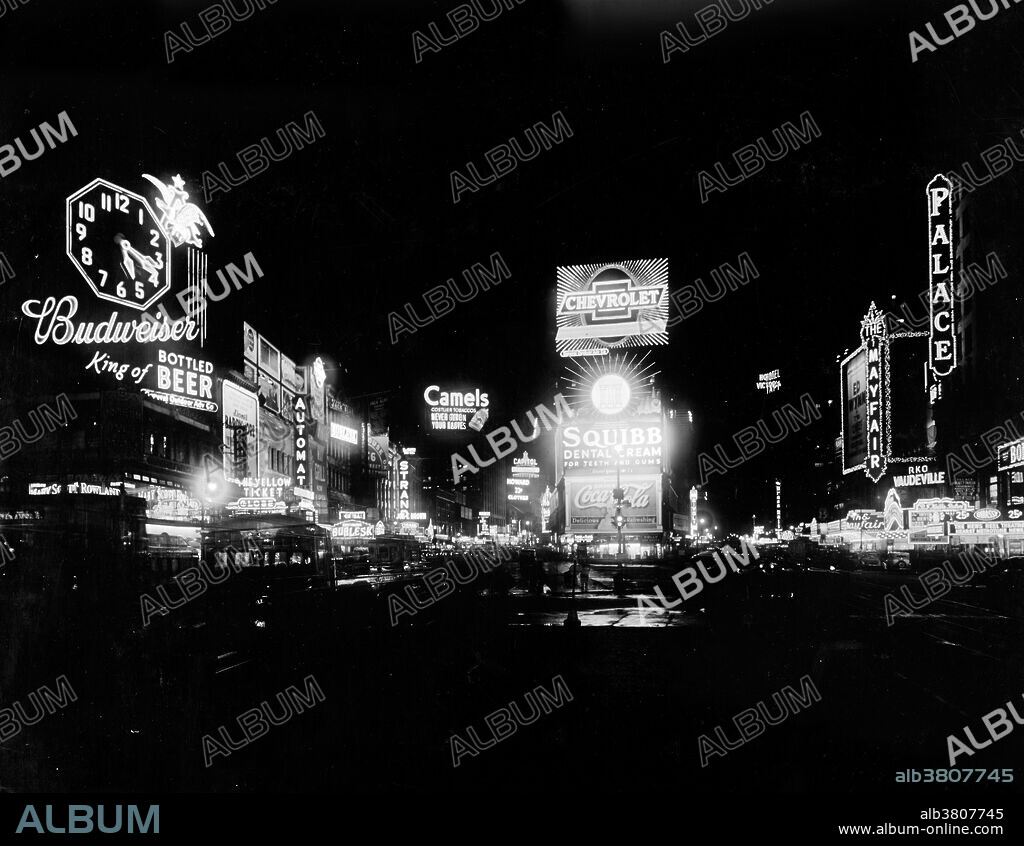The black and white photograph, a stock image from AlbumOnline, showcases a vibrant night scene of an early to mid-1900s city street brimming with neon advertisements. The image, rectangular with a longer horizontal edge, prominently features repeated watermarks of the word 'ALBUM' at a diagonal angle to prevent unauthorized use. Among the illuminated signs are advertisements for various products and establishments, including: Budweiser King of Bottled Beer, Camel cigarettes, Coca-Cola, Squib Dental Cream, Chevrolet automobiles, and theaters named Mayfair and Palace. Notable details include a clock above the Budweiser sign and a possible cowboy figure. The bottom right corner of the image displays the website www.album-online.com along with a code ALB 38 07745 repeated twice. The bustling nightlife depicted, reminiscent of modern Times Square, captures the era's lively urban atmosphere.